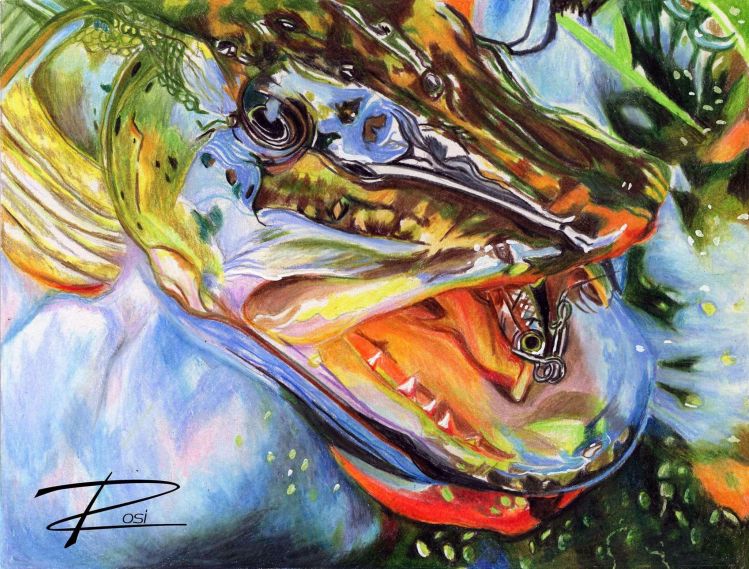This vibrant and abstract painting, likely created by an artist named Rosy, showcases a colorful and dynamic depiction of a creature's head, reminiscent of an alligator or dinosaur, with its mouth wide open. The artwork features a fiery palette of red, orange, yellow, green, blue, purple, and brown hues, blending seamlessly to create a sense of movement and vitality. The creature's black, shiny eye and sharp white teeth amplify its lifelike quality, while hints of blue suggest splashes of water, enhancing the dynamic scene. Inside the open mouth, there appears to be a metallic object resembling a fish or fishing lure, which adds an intriguing, almost surreal element to the piece. The signature "Rosy" in the bottom left corner confirms the artist's identity, stylized in a unique font that complements the painting’s eclectic style.